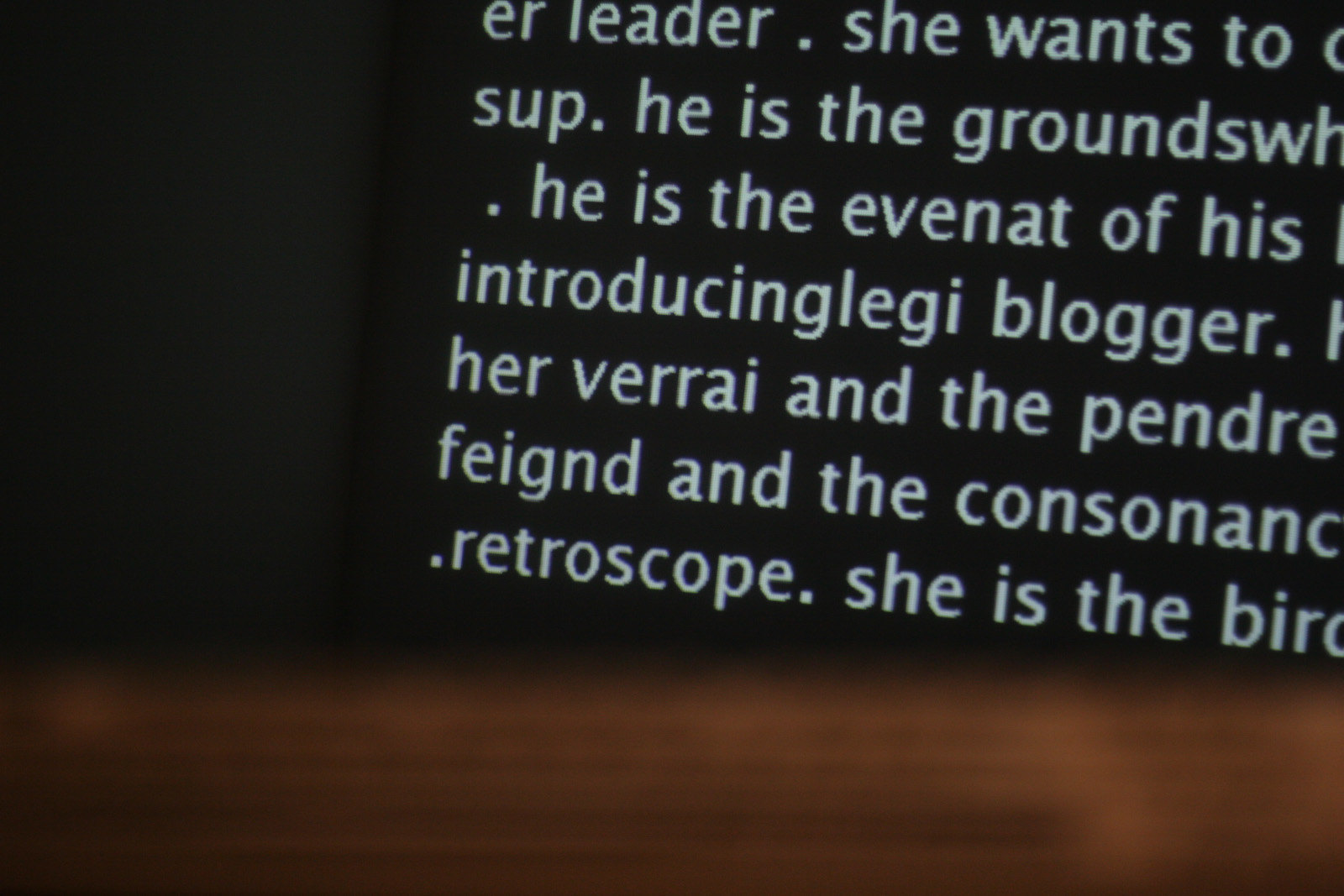The image shows a partially obscured excerpt from a story displayed on a digital device, possibly a Kindle or cell phone. The background is black, and the text is in white, creating a high-contrast effect that emphasizes the text as the focal point. The excerpt reads: "She wants to sup. He is the ground. He is the event of his introducing leggy blogger. Her veret in the pendre. Seined in the consonants retroscope. She is the bird." However, some words are cut off, making the text incomplete and somewhat cryptic. Along the bottom of the image is a blurry brown wooden border, which is not the focus but adds an additional element to the visual composition.